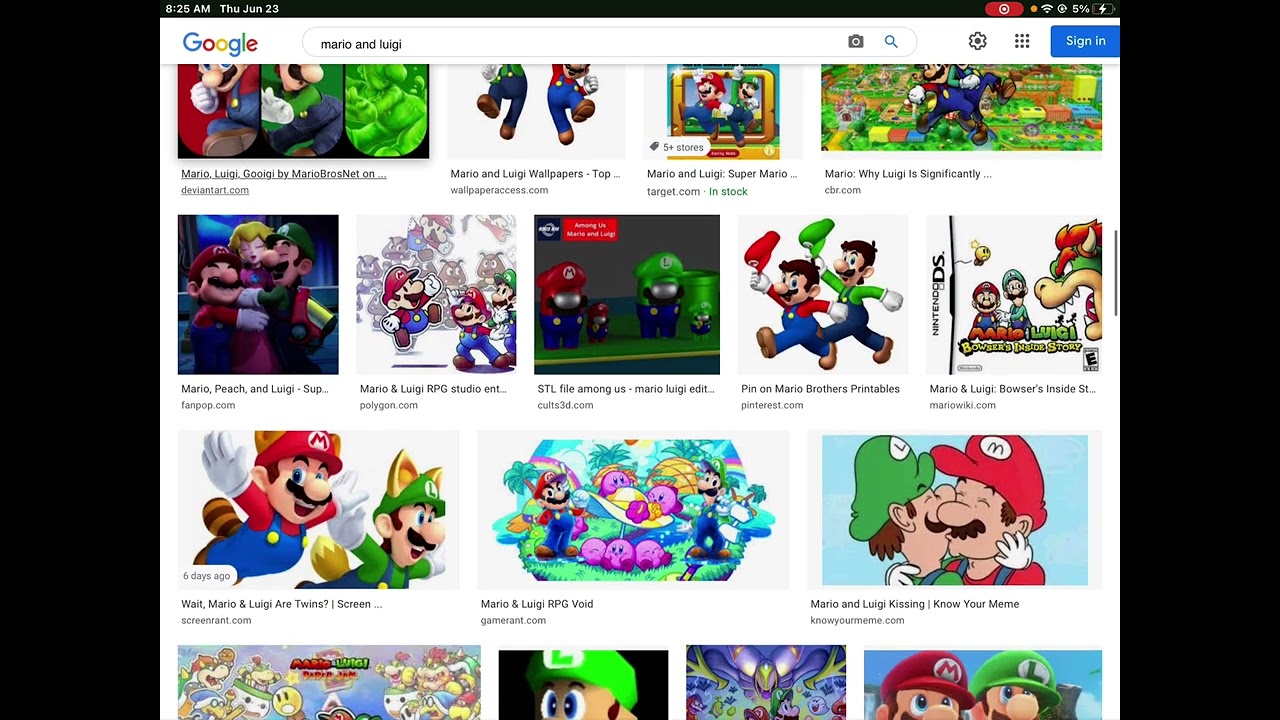The image in question appears to be a screenshot taken from a smartphone featuring a predominantly black background. At the very top left corner, the time is indicated as 8:25 AM, coupled with the date, Thursday, June 23rd. Adjacent to the time, there is a peculiar red oval symbol encompassing a white circle with a central white dot, likely a notification or app icon. To the immediate right of this icon, there is a Wi-Fi signal indicator, followed by a nearly depleted battery icon, showing just 5% charge.

Beneath this header, the screenshot transitions to a white background. In the upper left corner, the word "Google" is displayed next to a search bar, in which the phrase "Mario and Luigi" has been typed. To the right of the search bar, there is a photo icon accompanied by a magnifying glass, and further right, a blue "Sign in" button is visible.

Below this search interface, the screen is populated with an array of Mario and Luigi images. These are organized in four horizontal rows. The first row contains four images, the second row holds five images, the third row presents three images, and the fourth row, which is slightly cut off at the bottom, shows four images. The images are clearly aligned in a grid layout, illustrating various depictions of the iconic video game characters, Mario and Luigi.